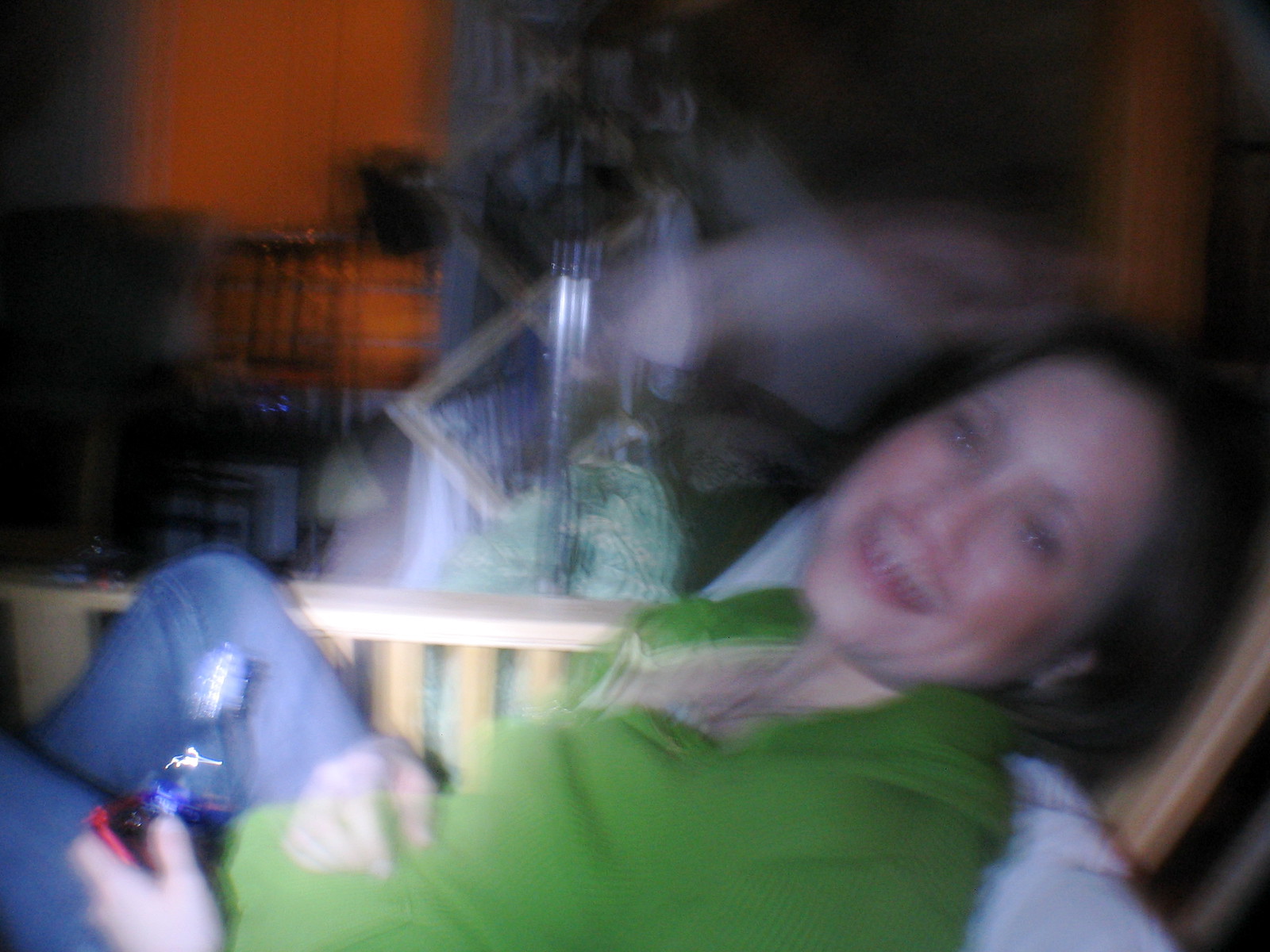In this very blurry photograph, a young woman is seen sitting and leaning back in a natural wooden chair with a light-colored pillow behind her. She appears to be laughing, as her head is turned to the side, revealing her smile and visible teeth. She has fair skin, dark brown hair, and is wearing a lime green collared shirt paired with jeans. Her face is accentuated with eye makeup, lipstick, and some blush, giving her a radiant look despite the blur.

Her left hand is holding an indeterminate bluish object, possibly a water bottle, while her right hand rests on her stomach. One of her knees is up and the other is down. The background is significantly out of focus, rendering it difficult to discern specific details, though it appears to be cluttered with various objects. These include a black-capped silver pole, possibly part of another piece of furniture, and a mix of items piled high, alongside what seems to be a red wall and some cloth in shades of green and yellow. The overall scene suggests it is nighttime, illuminated primarily by camera flash, with a lamp possibly glowing faintly in an adjacent room.